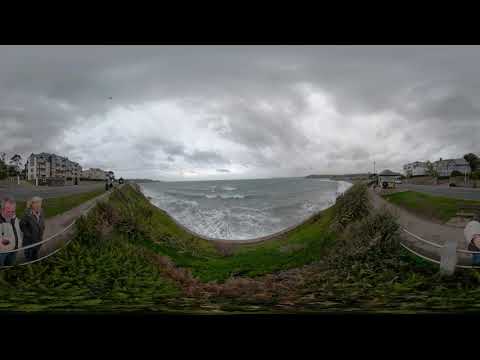The image captures a wide-angle, fisheye view of an overcast coastal scene on a stormy day. The gray, cloudy sky looms above, contrasting with the dark, choppy ocean water that breaks into foamy white waves against a green, grassy shoreline. In the foreground, a two-rail white fence separates a sidewalk from the turbulent beach, where an older couple, dressed in jackets and long sleeves, stands gazing at the waves. The grassy area lines either side of the water inlet, bordered by roads that stretch towards residential and commercial buildings. On the far right, several white houses are visible, while on the left, multi-storied structures, possibly hotels, overlook the unsettled ocean. The overall atmosphere suggests a cold, windy, and somber day by the sea.